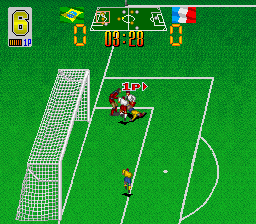The image is a still from an old-fashioned digital video game, likely of a soccer match, featuring a pixelated bright green grass turf field. Prominently displayed on the left is a large white soccer goal net. At the top of the image, the scoreboard shows 3 minutes and 28 seconds left in the match, with both the Brazilian team on the left and the French team on the right having a score of 0-0. A number "6" is also visible in the top left corner. The game's interface includes detailed white lines marking the soccer field and small character sprites representing the players. The Brazilian players, in yellow uniforms, and the French players, in white and red uniforms, are positioned on the field with a soccer ball in play, suggesting impending action in the game.